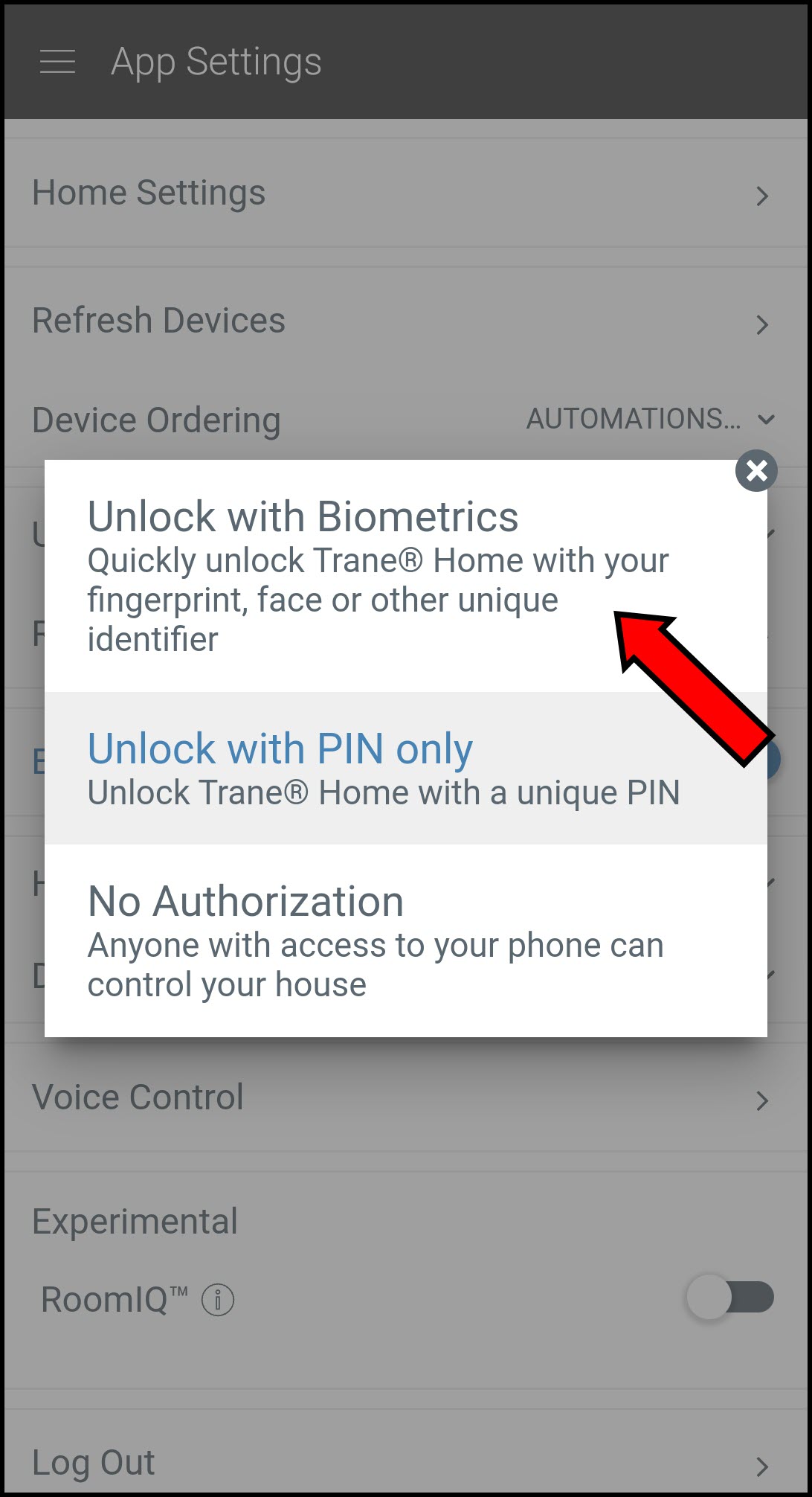The image depicts a mobile screen interface with a gray background, prominently featuring a white, pop-up section in the center. The pop-up is divided into three distinct sections. The top section is highlighted with a red arrow, outlined in black, pointing towards it. This section is labeled "Unlock with Biometrics" and provides information stating, "Quickly unlock Train Home with your fingerprint, face, or other unique identifier."

Below this, in blue text, is the second section labeled "Unlock with Pin Only," which explains, "Unlock Train Home with a unique pin or no authorization. Anyone with access to your phone can control your house." At the top right corner of the pop-up, there's an 'X' icon to close it.

In the main gray background of the screen, various app options are listed. At the top, it says "App Settings," followed by "Home Settings," "Refresh Devices," "Device Ordering," "Automations," "Voice Control," and "Experimental." Additionally, there is an option labeled "Room IQ" with a toggle button, which is currently toggled off. Below these settings, there is a "Log Out" option. The entire screen is encased within a slight black border.